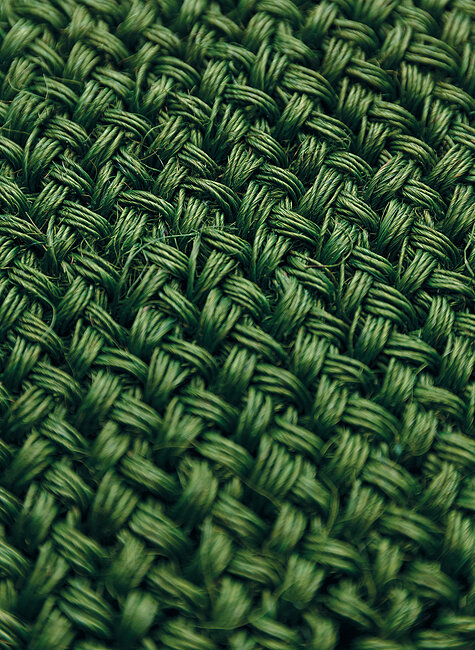This extreme close-up photograph showcases the intricate details of a knitted green fabric. The zoom level reveals individual threads forming a crisscross pattern by looping into one another, creating a larger, cohesive textile. The fabric, captured at a slight angle from top left to bottom right, presents a uniform stitching method, although occasional frayed strands and minor wear spots disrupt its consistency. In the center, clusters of five threads band together, illustrating the common practice of aggregating multiple threads for added thickness. The image prominently features eight vertical rows weaving through the frame: the far left row partially visible at the top, six central rows extending off the image at various angles, and the final row peeking from the upper right corner. Despite the meticulous structure, some threads appear ever so slightly frayed or loose, hinting at gentle wear or usage over time.